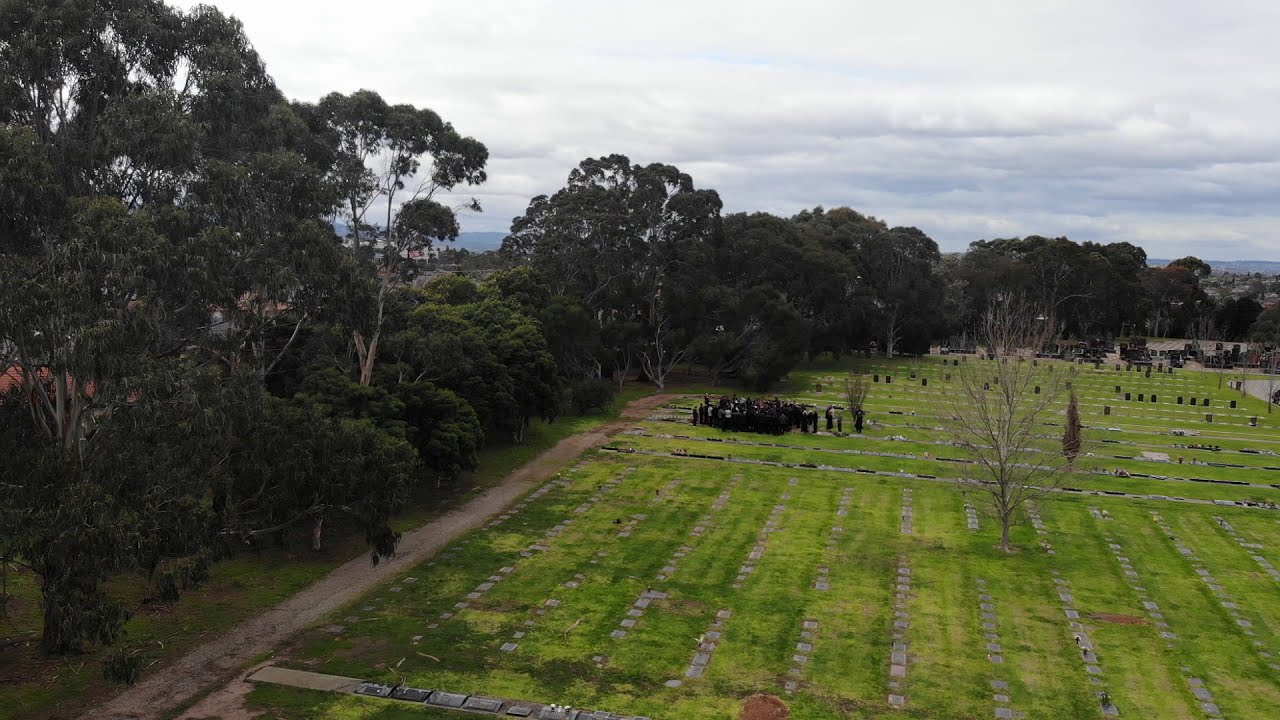From a high vantage point, the image depicts a somber cemetery scene under a gray, cloudy sky. The expansive green field is dotted with rows of flat, rectangular grave markers arranged in orderly lines. A dirt road, bordered by greenery, winds along the left side of the cemetery, enclosing the rows of markers. In the center of the image, a large cluster of people dressed in black—a funeral procession—gathers near a solitary, leafless tree. Off in the distance, darker, more prominent headstones are visible, standing tall among the flat markers. Scattered around the area, there are trees with lush green leaves, providing a contrasting backdrop to the gray headstones and the grieving crowd. A building can be faintly seen far off, adding to the depth of the image. Additional figures are seen walking up the road towards the group of mourners, adding a sense of movement to this somber tableau.